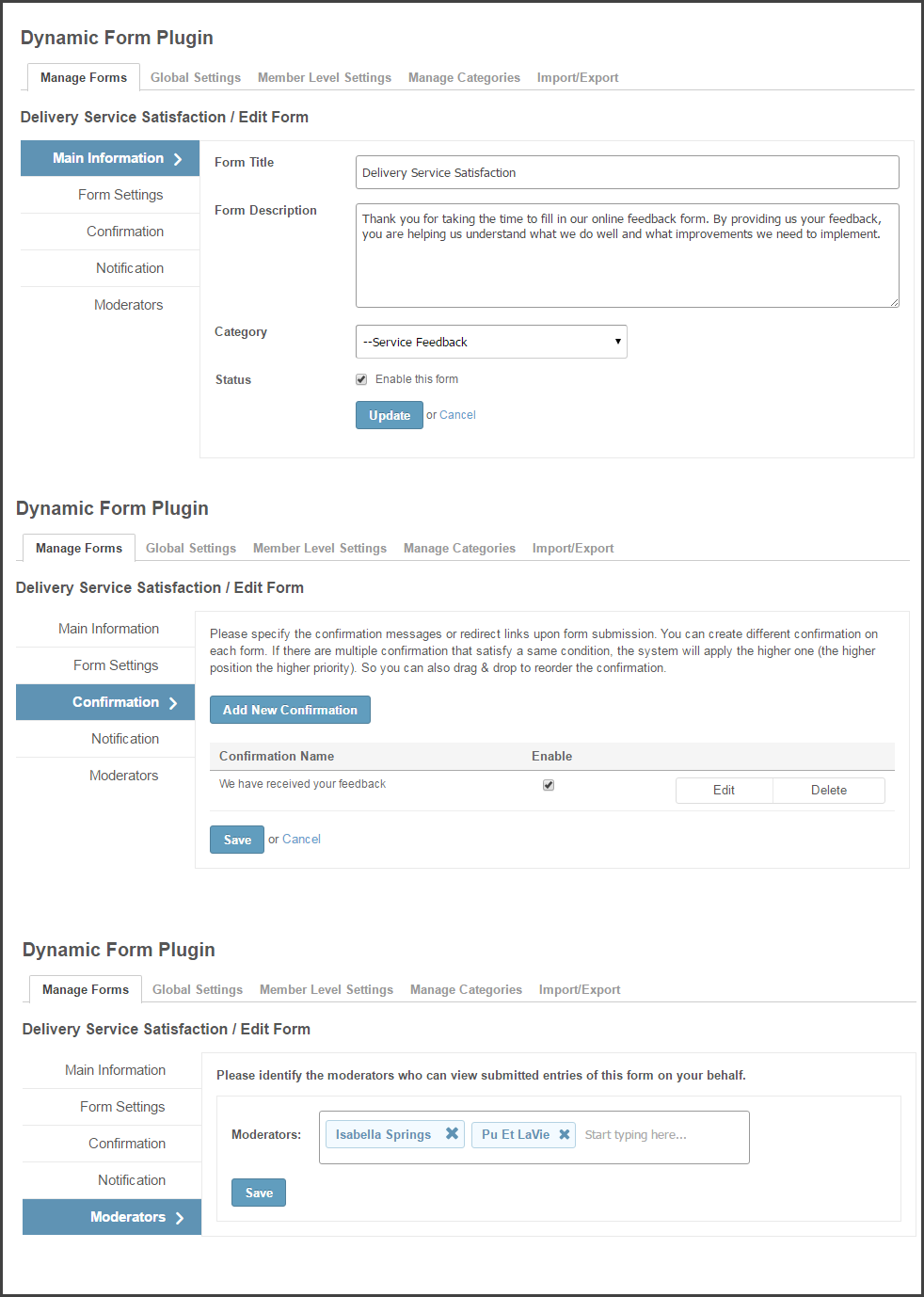The image displays a technical page for a "Dynamic Form Plugin" with multiple options available in the header, including "Manage Forms," "Global Settings," "Member Level Settings," "Manage Categories," and "Import/Export." The current focus is on "Manage Forms," showcasing a form titled "Delivery Service Satisfaction." This form aims to gather feedback to help improve service quality.

The interface highlights "Main Information" with a blue button, and other options such as "Form Settings," "Confirmation," "Notification," and "Moderators" are also available. The page includes a description thanking users for their feedback, stating: "Thank you for taking the time to fill out our online feedback form. By providing your feedback, you are helping us understand what we do well and what improvements we need to implement."

Additionally, there is a drop-down menu enabling selection for service feedback and buttons to enable the form, update, or cancel it. Below this, another similar form section appears, but this time, "Confirmation" is selected instead of "Main Information." It prompts users to specify various details. The page exemplifies different configurations within the "Delivery Service Satisfaction" form under the "Edit Form" section.